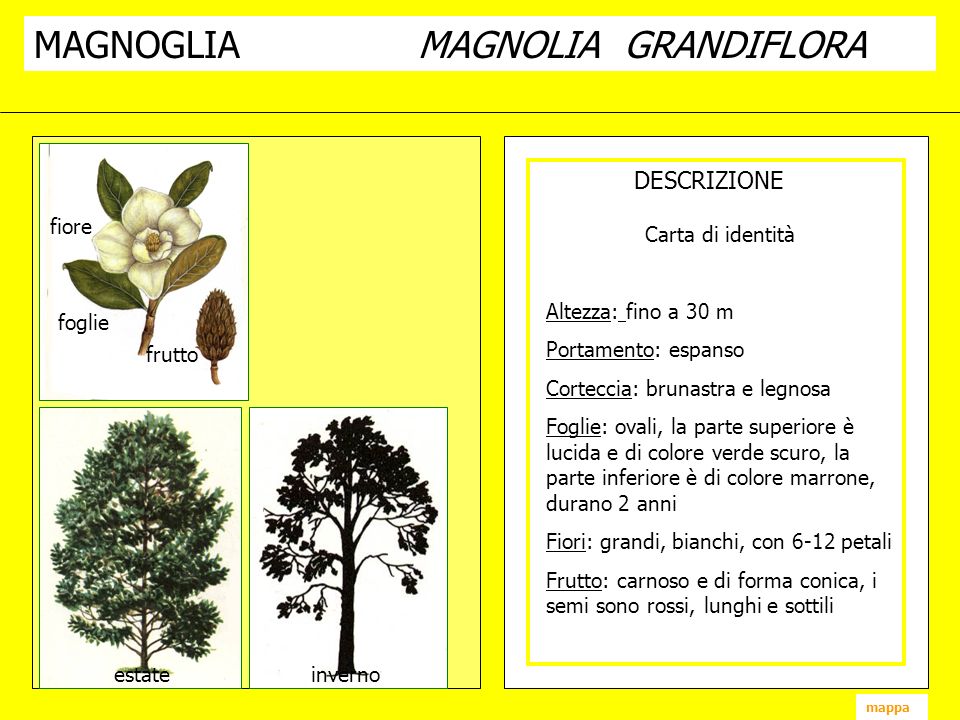The image presents a detailed, educational poster primarily titled "Magnolia," with "Magnolia Grandiflora" in italics underneath, all against a white strip at the top. Below this, the background transitions to yellow and is sectioned into two main parts: the left and right. 

On the left, there is a square arrangement of three images. The top image is a close-up of a Magnolia Grandiflora flower, showcasing cream-colored petals with dark green leaves, labeled in a foreign language as "Fiore, Fogli, and Fruto." The middle image depicts a green-leaved tree marked "Estate," indicating its summer state. The bottom image portrays a bare black tree labeled "Inverno," symbolizing its winter state. 

The right side of the poster is filled with extensive text, which appears to be an informative description in what looks like Italian. This text includes headings like "Descripcion Carta de Identidad" and covers specifics such as "Alteza, Fino A30M, Portamento Esponzo, Corteccia Brunestra e Laginosa," detailing the plant's height, spread, bark, and more. The meticulous layout contrasts the visual representations on the left with the descriptive content on the right, providing a comprehensive overview of the Magnolia Grandiflora species.